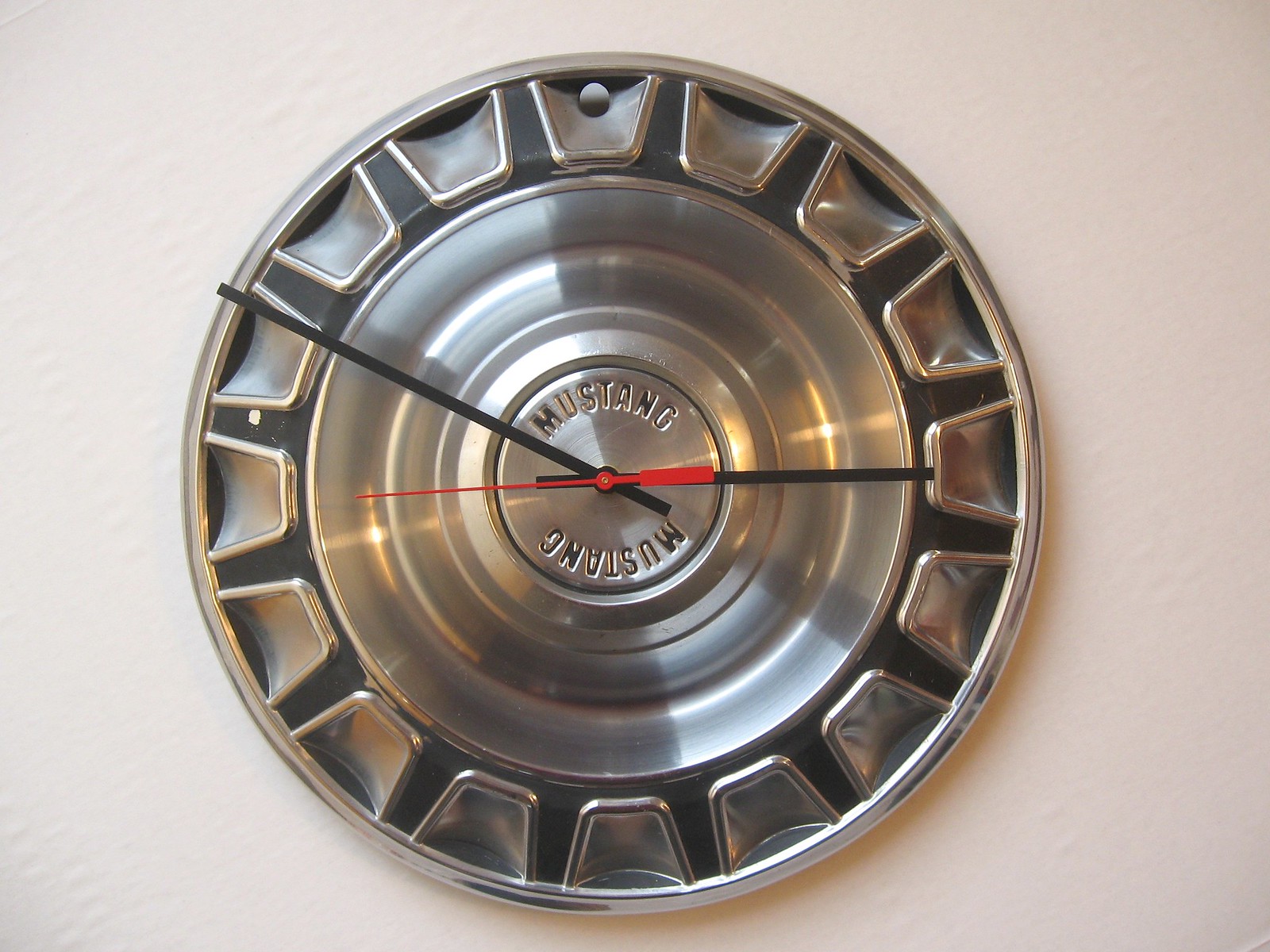An indoor, close-up photograph showcases a uniquely crafted wall clock mounted on a white wall. The clock's face is an authentic-looking reproduction of a Mustang hubcap, likely reminiscent of designs from the 1960s. It is meticulously crafted from stainless steel, gleaming under the light. The absence of numerals on the hubcap does not detract from its distinctiveness, as the time is indicated by sleek black hour and minute hands and a red second hand, which currently points to the 9. The hour and minute hands are positioned to show a time of approximately 2:50.

At the center of the hubcap, a Mustang emblem proudly displays, encircled by the word "Mustang" in bold black letters at both the top and bottom. An original touch is the presence of a single hole located at what would be the 12 o'clock position, likely where the air nozzle would have protruded if it were still functioning as a hubcap. The pristine condition of this hubcap suggests it might be a new reproduction, creatively repurposed to serve as a wall clock. The minimalist yet distinctive design offers a perfect blend of vintage automotive charm and contemporary home décor.